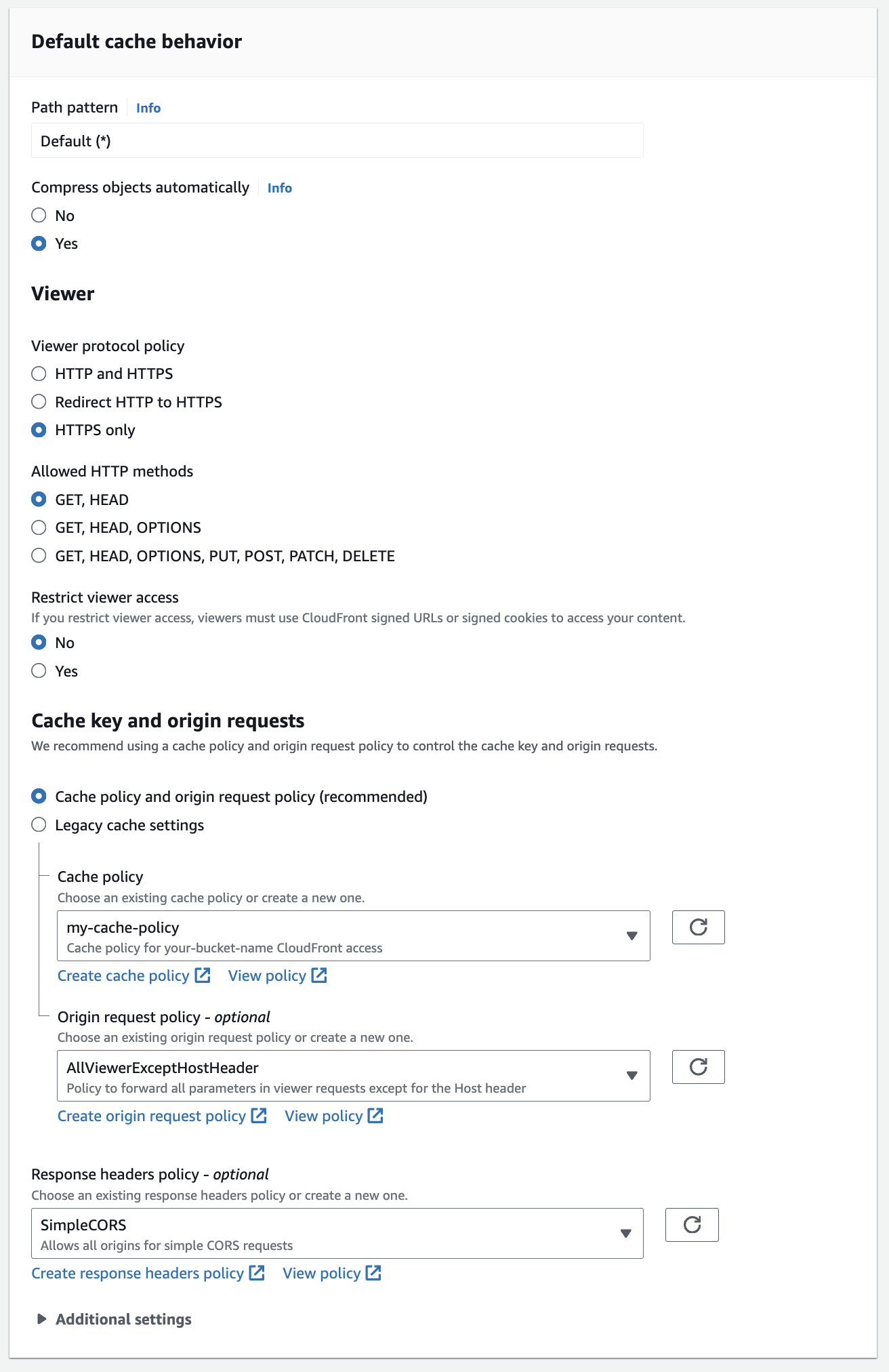This image captures a detailed configuration screen for setting a default cache behavior. 

At the top, the section labeled "Path Pattern" is visible, with a blue "info" icon to its left. Underneath this section, the word "Default" is displayed.

Further down, there's an option labeled "Compress Objects Automatically". To the left of this text, another blue "info" icon is present. Next to this option, there are two radio buttons labeled "No" and "Yes." The "Yes" option is selected, indicated by a blue circle with a white center.

Beneath this, there is a section labeled "Viewer Protocol Policy" with three options: "HTTP and HTTPS," "Redirect HTTP to HTTPS," and "HTTPS Only." The "HTTPS Only" option is selected.

Going further, the screen displays options such as "Allow HTTP Methods," "Restrict Viewer Access," and a comprehensive section titled "Cache Keys and Origin Requests," which includes various selectable options.